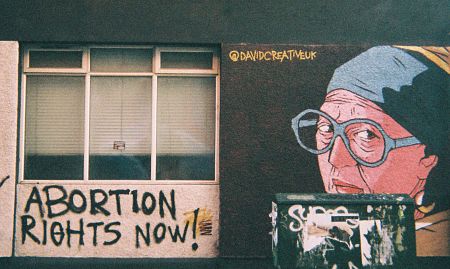The photograph captures a color image of an outdoor scene featuring the side of a stucco building bathed in natural light. The horizontally rectangular image presents a detailed mural and graffiti on a light brown wall. Three rectangular windows are seen on the left, each adorned with horizontal sections and partially lowered Venetian blinds, leaving about 20% of the bottom black. In bold black spray paint beneath the windows, the message "Abortion Rights Now!" is vividly inscribed.

On the right side of the image, a mural dominates the scene, featuring an older woman adorned with thick, round blue glasses, an earring, and a blue bandana covering her blonde hair. This mural is signed in gold in the upper left corner as "David Creative UK." Positioned in front of the mural is a green dumpster with white graffiti, aligning just below the woman's lips in the artwork and extending down to the ground. The combined elements of the mural, graffiti, and windows create a compelling and layered visual narrative on the building's wall.